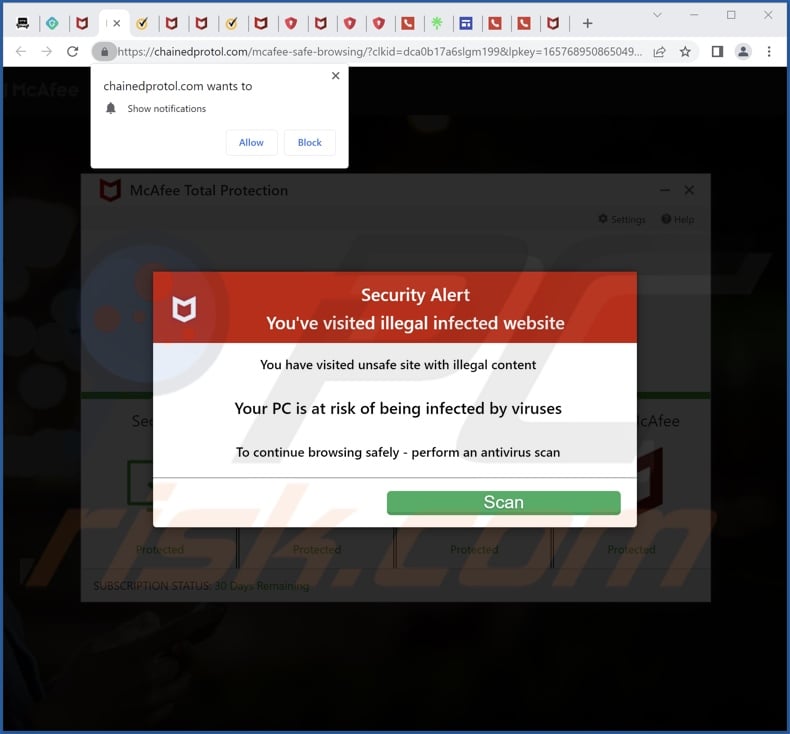This image is a detailed screenshot of a website, specifically chainedprotocol.com, showcasing multiple security-related pop-up boxes. The most prominent pop-up is a red and white alert box with a green scan button, warning the user that they have visited an unsafe site with illegal content, putting their PC at risk of being infected by viruses. It advises performing an antivirus scan to continue browsing safely. 

At the top of the screen, various notifications and icons appear in multiple colors including red, green, blue, white, black, yellow, and orange. Another pop-up from chainedprotocol.com requests permission to show notifications, offering "Allow" and "Block" buttons.

In the background, behind the security alert pop-up, is a McAfee Total Protection interface, displaying settings and help buttons. Text on the interface includes messages like "protected" and "subscription status," indicating that the McAfee subscription has 30 days remaining.